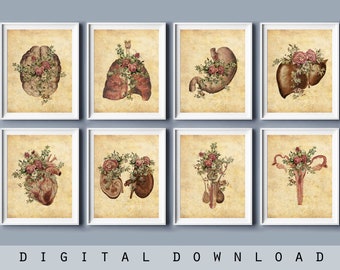The image showcases a product with a dark gray background featuring eight white-framed pieces of artwork arranged in two rows of four. Each individual frame contains an anatomical human organ illustration set against a vintage, light brown (or beige) background. These organs are creatively depicted with flowers emerging from them, giving each piece a distinctive and artistic appearance. The organs include a brain, lungs, stomach, liver, heart, kidneys, male genitalia, and female genitalia (including the uterus). At the bottom of the image, a light gray banner with black capitalized text reads "DIGITAL DOWNLOAD," indicating that the artwork is available for digital purchase.